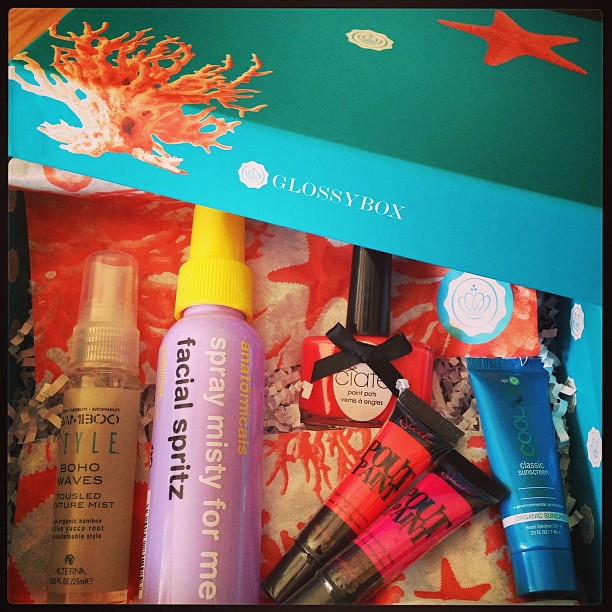The image depicts an open turquoise and green gift box adorned with sea creature and coral illustrations, and the text "Glossy Box" in white. Inside the box, nestled amidst red and white tissue paper, are several self-care and beauty items. On the left, there's a beige bottle labeled "Boho Waves Tasseled Moisture Mist." Next to it, a purple bottle with a yellow spray cap reads "Anatomicals Spray Misty for Me Facial Spritz." A red bottle of nail polish labeled "Ciate" features a black bow. Additionally, there are two lip products in tubes marked "Pout Paint"—one in deep orange and one in bright pink. Finally, on the right side of the box, a blue squeezy tube labeled "COOLA Classic Organic Sunscreen" completes the collection.